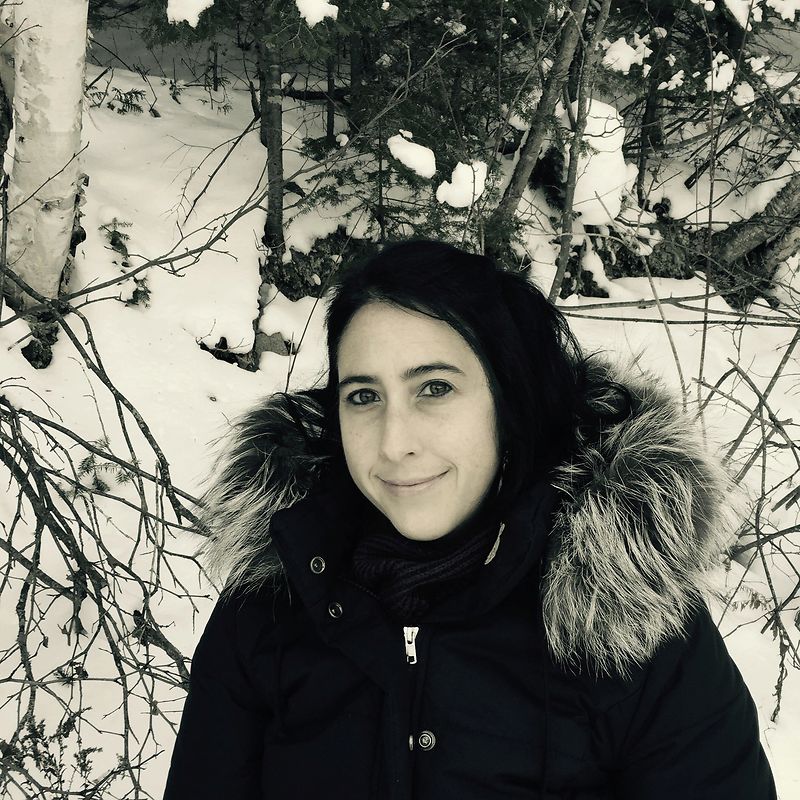In this square-format photograph, a young woman in her 20s stands against a wintry backdrop, gazing up at the camera with a soft smile and dark, hazel eyes. Her black hair contrasts with her pale, slightly tinted skin. She wears a black, zip-front coat adorned with a large fur collar that encircles her neck and shoulders, featuring fur with black and crystal tips. The outdoor scene is blanketed in snow, with large trees and numerous branches forming a stark, leafless canopy behind her. The snowy landscape includes clumps of snow on the branches and a slight hillside visible on the upper left side of the image. The overall coloration of the photo leans towards monochromatic tones with subdued hints of color, emphasizing the serene yet cold winter environment.